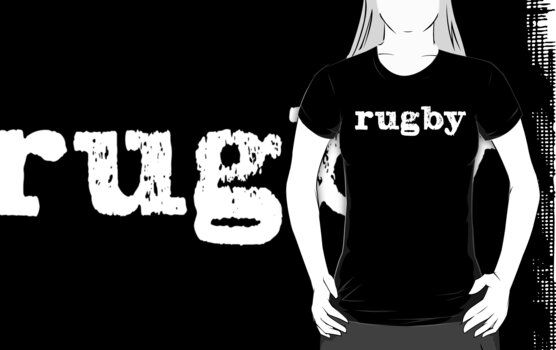The advertisement features a detailed sketch of a young woman standing confidently with her hands on her hips, showcasing a short-sleeved black rugby t-shirt with rugged white text that reads "rugby." The woman, depicted in a minimalist cartoon style, has white skin and long gray hair, donning a pair of gray pants. The monochromatic background presents a grunge aesthetic, predominantly black with areas where light peeks through, resembling a worn tarp or cracked wood. Behind the woman, partially obscured, the word "rugby" is repeated in the same distressed white font, with only the initial letters "R," "U," and "G" clearly visible. To her right, a crisscross pattern in black and white further enhances the edgy, textured look of the advertisement.